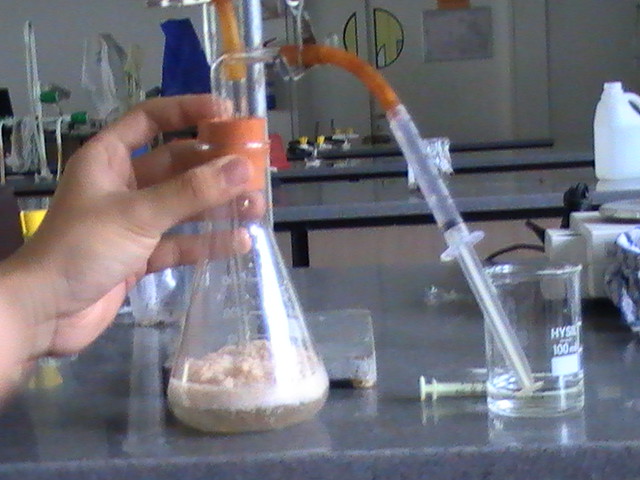The photograph appears to be taken inside a dimly lit science laboratory classroom with four rows of tables featuring gray granite tabletops and black frames. Dominating the center of the image is a youthful hand holding a flask or beaker. The flask, which has an orange cork in its top, contains an amber-colored liquid at the bottom, topped by a layer of foam. A rubber tube protrudes from the cork, connected to a syringe. This detailed setup suggests a lab experiment in progress, possibly an extracurricular activity. In the background, there are additional lab tables with various chemical containers and measuring equipment scattered nearby. Farther back, a sink with multiple glass displays and a large tub filled with liquid can be seen on a brown table. The scene gives an impression of a solitary student meticulously conducting an experiment in an otherwise empty classroom.